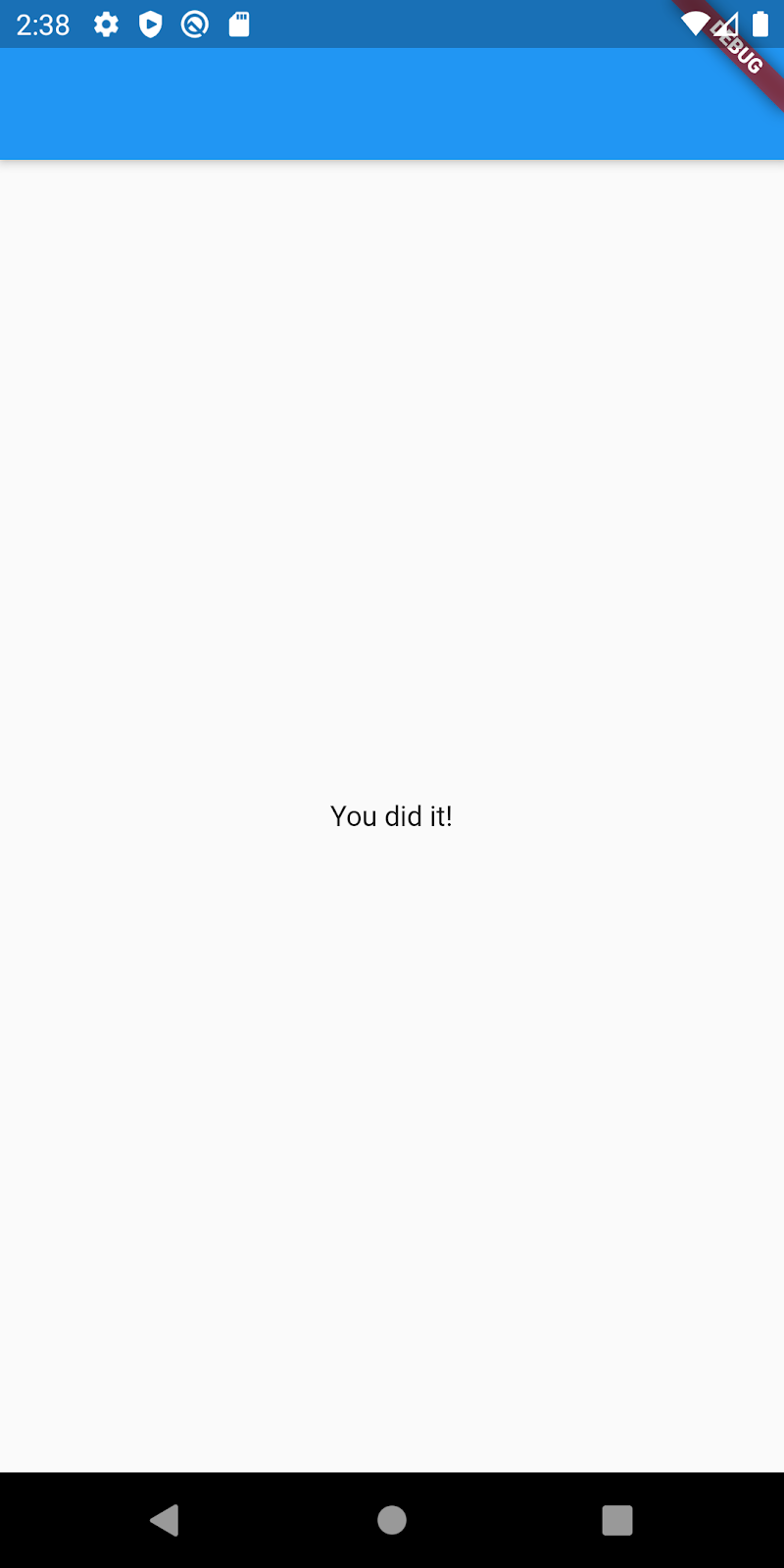The image showcases a screenshot likely taken from an Android device, as indicated by the user interface elements at the top of the screen. At the very top, there is a dark blue banner featuring several icons: "238" on the top left, followed by a cogwheel (possibly for settings), a shield with a play symbol, and another circle icon with an unclear detail inside. On the right side of the same banner, there are icons for WiFi (fully filled), signal strength (about half full), and a fully charged battery. Overlaying this section is a red-angled label with the text "debugged."

Below the dark blue banner, there is a thicker light blue banner that contains the congratulatory message "You did it" centered in the middle, with a lighter gray background. At the very bottom of the screen, a black banner houses three icons: a play symbol, a circle, and a square.